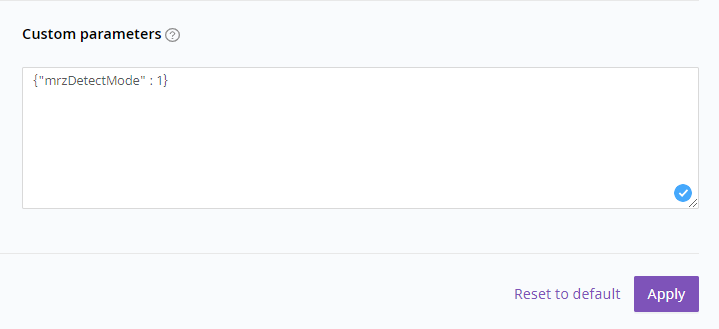This is a cropped screenshot capturing the "Custom Parameters" section of a form or settings interface, set against a light blue background. In the top left corner, "Custom Parameters" is prominently displayed in bold black font, accompanied by a gray question mark icon to its right, likely serving as a tooltip or help icon. 

Dominating the center of the screenshot is a large, rectangular white box containing a snippet of code. Within this code, the term "MRZ detect mode" is clearly visible. A blue circle with a white check mark is situated in the bottom right corner of the white box, signifying a successful validation or selection.

At the bottom right of the screenshot, "Reset to Default" is written in purple font, offering a reset option. Adjacent to this is a small purple button labeled "Apply" in large white font, designed for users to apply the custom parameters. At the very top of the image, a thin gray line from the section above, which was cropped out, is faintly visible.